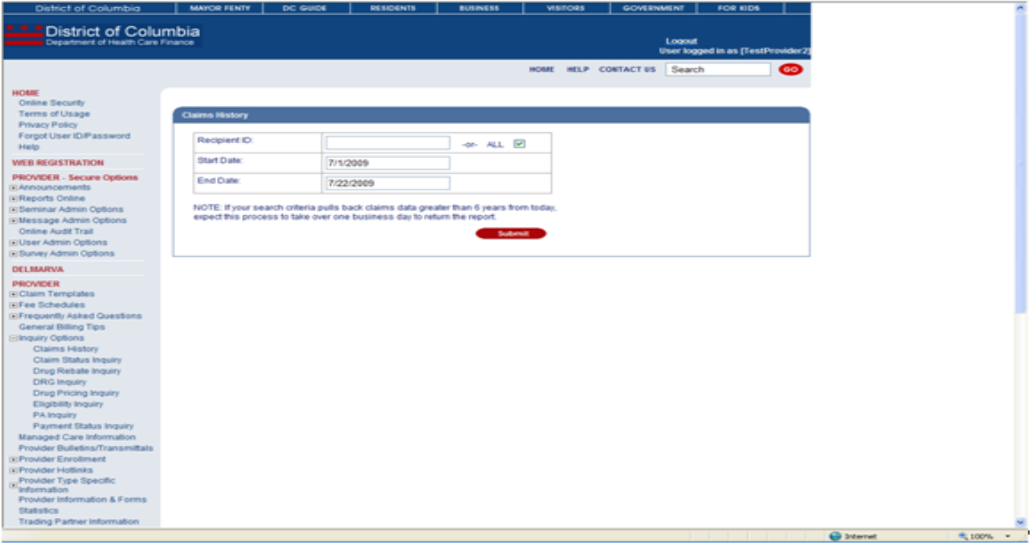The image appears to be a screenshot of a computer screen featuring a data management or registration interface. The interface has a distinctive blue background that spans from the left side of the screen to almost the far right. On the left side, there are two vertical red lines with three red dots at the top, adjacent to the text "District of Columbia."

A sidebar on the left contains several labeled sections: "Home," "View Registration," "Provider Secure Options," and another "Provider" section, each demarcated by a border. In the main area of the screen, there is a rectangular popup, which seems to be a selection menu with the header "Choose," possibly related to a historical data query.

Within this popup, there are fields for entering search criteria, including "Participant ID," "Start Date," and "End Date." The start date entered is 07-05-2009, and the end date is 07-22-2009, indicating the user is conducting a search for participant records within that timeframe.

The lower portion of the screen is predominantly white, providing a clean background for additional information that might be displayed upon executing the search. The right and bottom edges of the screen also feature white space, adding to the uncluttered appearance of the interface.